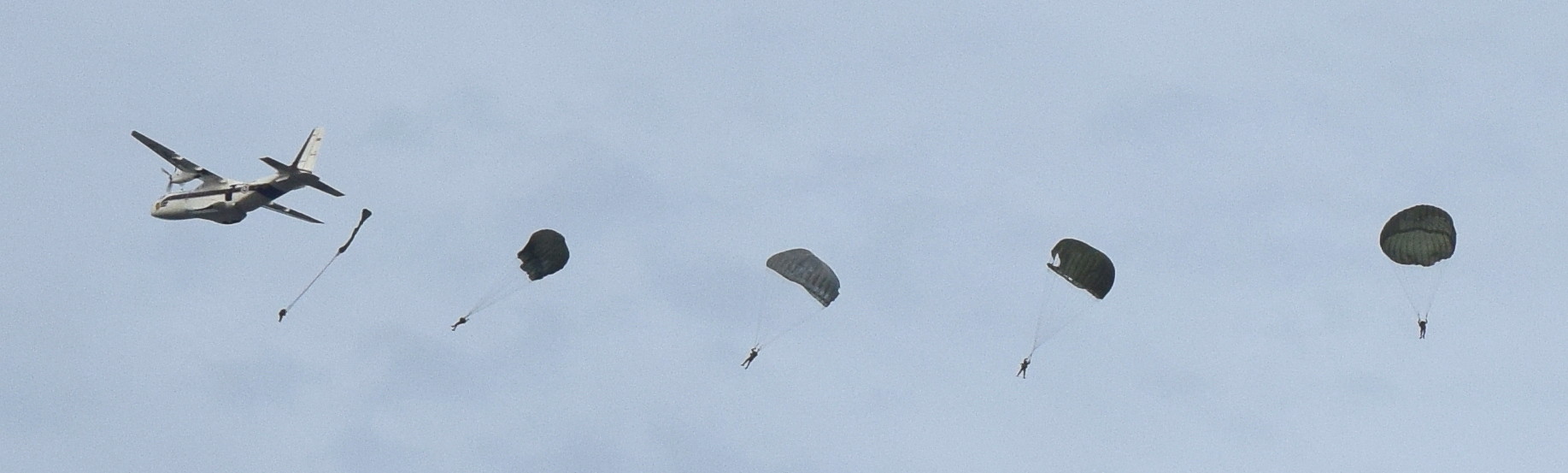The photograph, a very narrow landscape orientation, captures a vivid skydiving scene against a blue sky dotted with clouds, taken from the ground and zoomed in. On the left side, a propeller airplane is flying away to the left, with only its side and back visible. Emerging from the back of the aircraft are five parachutists in various stages of their jumps. The skydivers are dispersed from left to right across the sky, with their parachutes at different stages of deployment.

The closest parachutist to the plane's rear has just jumped out, and their parachute appears as a barely discernible thin line. The second parachutist has a parachute starting to open, creating the initial concave shape. Moving further right, the third and fourth parachutists have their parachutes partially opened, showing more of the mushroom cap shape. The fifth and farthest parachutist has a fully deployed parachute, with clear thin strings and a tiny silhouette figure of the jumper visible. The parachutists' bodies appear tilted at angles due to the inertia from their initial leap out of the aircraft.